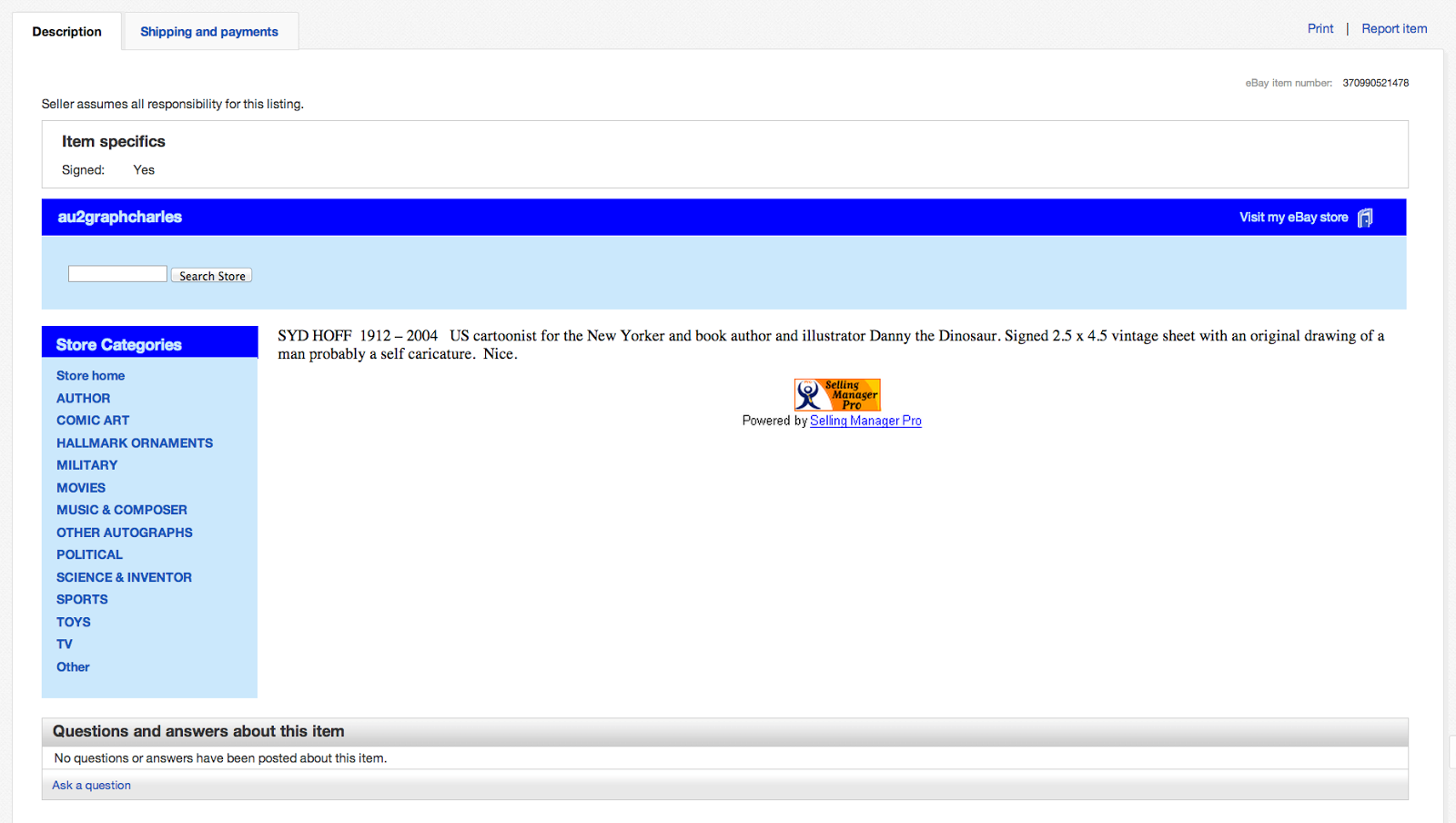In the center of the image, there is a prominent blue rectangle with a gradient transitioning from dark blue at the top to lighter blue at the bottom. Adjacent to this, there is a rectangular search box labeled "Search Store," where users can type in their queries. 

To the left side of the image, various store categories are listed: "Store Home," "Author," "Comic Art," "Hallmark Ornaments," "Military," "Movies," "Music and Composer," "Other Autographs," "Political," "Science and Inventor," "Sports," "Toys," "TV," and "Other." 

On the right side, gray text reads, "SYD HOFF, 1912 - 2004, U.S. cartoonist for The New Yorker and author/illustrator of 'Danny and the Dinosaur.' Signed 2.5 by 4.5 inch Vintage Sheet with an original drawing of a man, likely a self-caricature, and the word 'Nice.'" 

In the center, there is a small note indicating that the site is "Powered by Selling Manager Pro." At the bottom left of the image, there is an option labeled "Questions and answers about this item." In the very bottom left corner, blue text offers the option to "Add a question" by clicking on it.